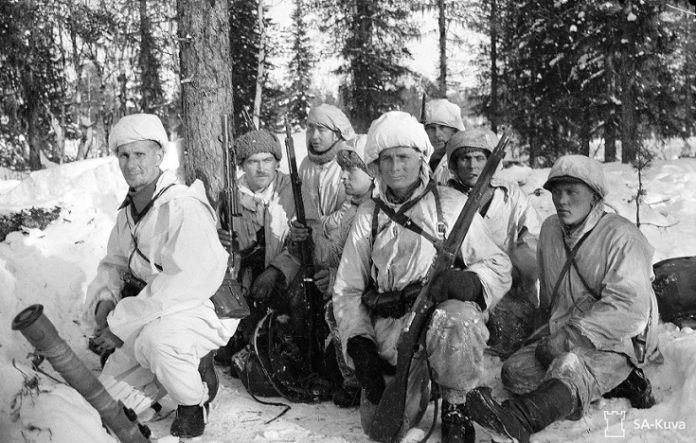This black and white photograph captures a group of eight soldiers, likely from an army unit, positioned in a snow-covered forest with pine trees in the background. The soldiers, dressed in winterwear with predominantly white or gray uniforms and Russian-style fur hats, are either kneeling or sitting on the snowy ground. Most of them are holding rifles, while the soldier on the far left is equipped with a rocket launcher or a similar large tube-like weapon propped in the snow beside him. The soldiers are looking in various directions, with one notable figure among them sporting a mustache. In the bottom right corner of the image, there's a photo credit marked "S-A-K-U-V-A" accompanied by a small chess rook symbol.